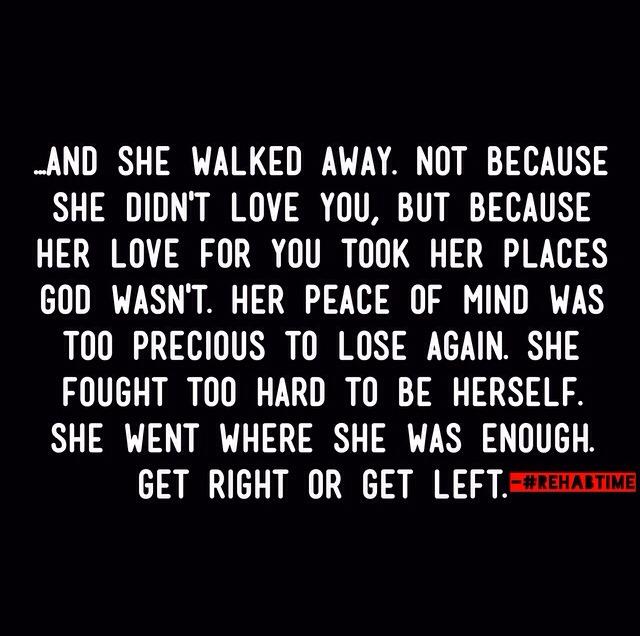The image features a stark black background with a poignant white message in all uppercase letters. The text reads, "...AND SHE WALKED AWAY. Not because she didn't love you, but because her love for you took her places God wasn't. Her peace of mind was too precious to lose again. She fought too hard to be herself. She went where she was enough. Get right or get left." In the lower right corner, a red banner contains the black text: "#REHASTIME". The entire design is clean and minimalist, focusing solely on the powerful quote without any other identifying marks or borders.